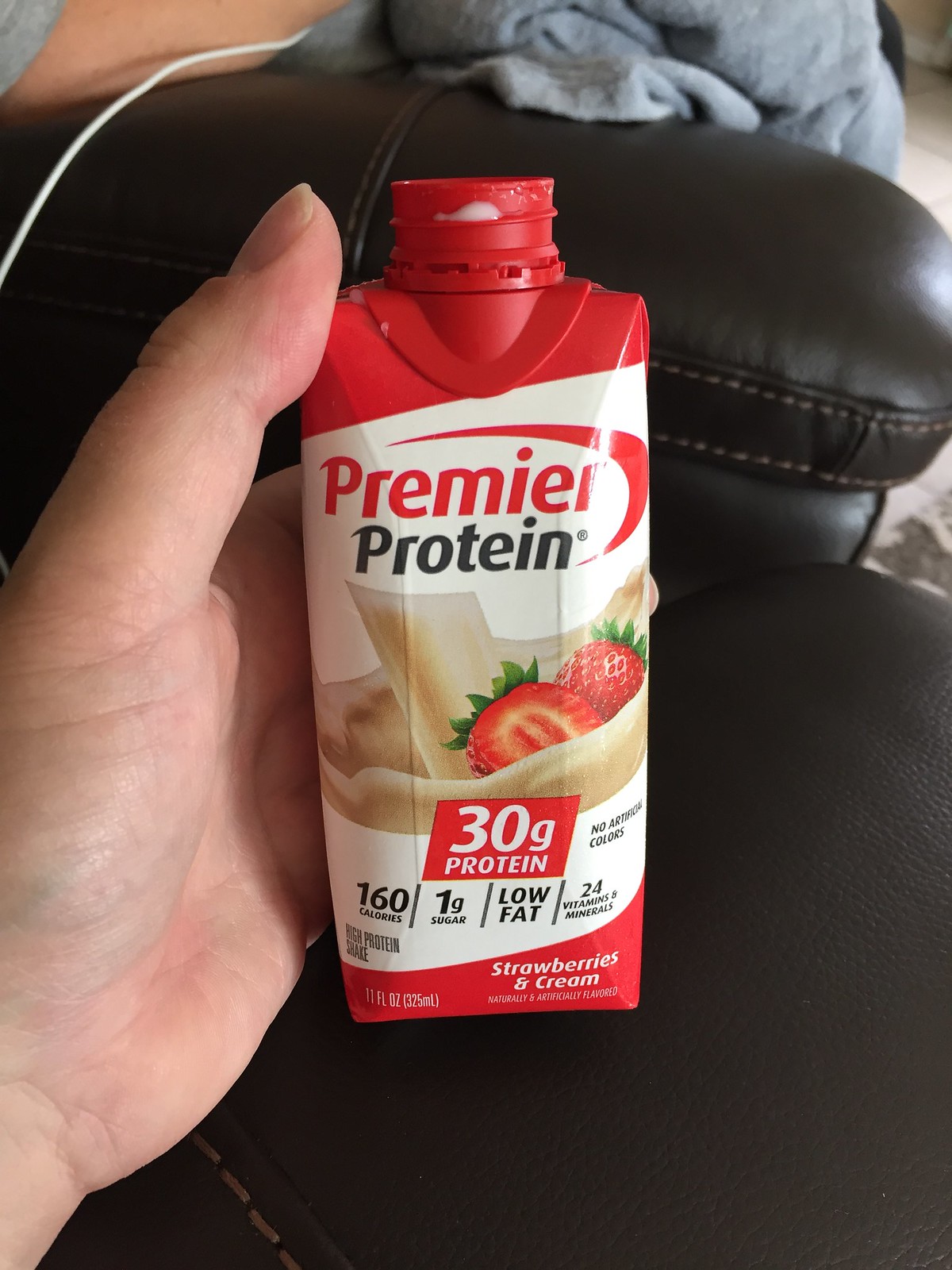The image showcases a close-up, indoor photograph of a Premier Protein drink in a small, square-like plastic carton being held by a person's left hand. The carton features a red round cap at the top, which has visible condensation and extends slightly over the side. The design of the carton includes a red top section, a white central section, and a thin red strip at the bottom. The white section prominently displays the text "Premier Protein" in black and is framed by a red semicircular shape. Below this, an image of the product is shown, with a milk splash and two strawberries—one sliced to reveal the inside and another whole strawberry in the background. A slightly tilted red rectangle above the image states "30g Protein" in white letters, followed by details like "160 calories," "1g sugar," "Low Fat," and "24 Vitamins and Minerals" in smaller text. The flavor description "Strawberries and Cream" is written in white text on a red background at the bottom right corner of the carton. In the background, the setting appears to be indoors with a glimpse of a black sofa or chair's armrest, part of a person's right elbow, a diagonal cord, and a light blue crumpled blanket or afghan. The image indicates that the person holding the drink has already taken a few sips, as there is a bit of the drink visible on the neck of the bottle.